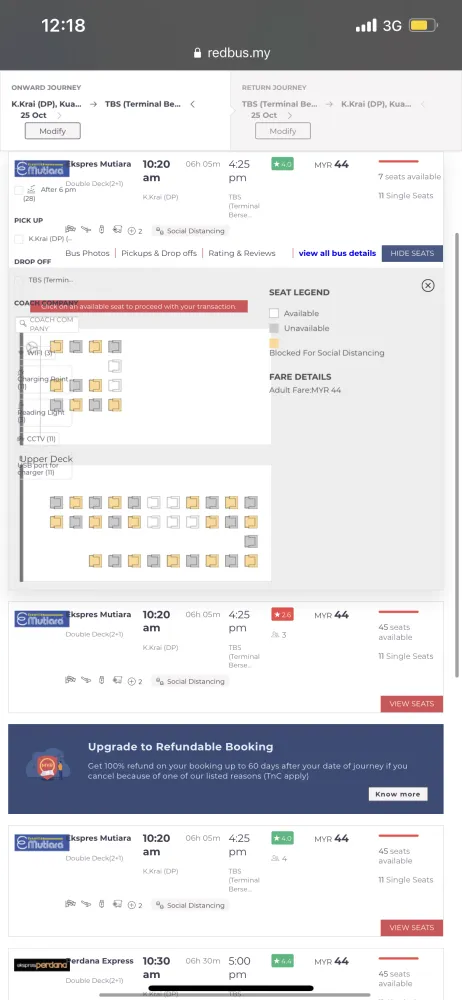The image is a vertical screenshot taken on a cell phone, depicting a flight seat map on the RedBus.my app. At the top, a gray banner displays the website address “redbus.my”. Below the banner, the flight route is marked as "DP to TBS", with options to modify the journey parameters positioned just beneath.

Further down, the display outlines the flight details, including both the arrival and departure times. Dominating the center part of the image is a large gray section that presents a seating map, allowing the user to select their seat. The seat availability is color-coded: available seats are marked in white, unavailable seats in yellow, and seats blocked for social distancing are marked in gray.

Below the seating map, additional flight details are provided. Immediately following is a dark blue banner with white text offering an "Upgrade to refundable booking" option, accompanied by a button labeled "No more".

At the bottom of the screen, two more flight detail boxes are shown, including two red buttons that invite the user to "View seats" for a specific part of the flight. In the upper left-hand corner of the image, the current time is displayed as 12:18. The upper right-hand corner shows a fully-filled signal indicator marked "3G" and a battery icon also fully charged, represented in yellow.